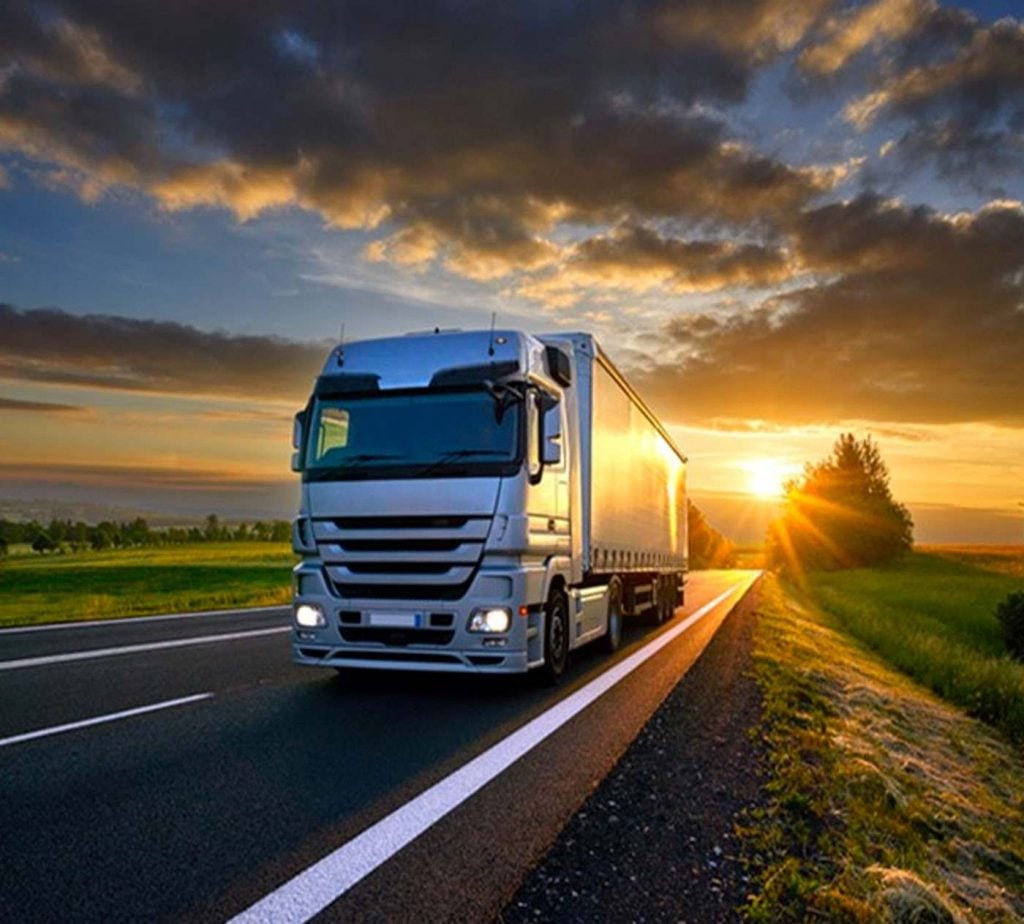The photograph captures a large, shiny, silver-colored semi-truck with its headlights on, pulling a long trailer down a clean, freshly asphalted two-lane highway, with an adjacent shoulder on the right side. The perspective is from the left lane as the truck approaches. The setting is rural, surrounded by expanses of tall grass fields on both sides of the highway, with trees visible in the distance and rolling hills or clouds on the horizon. The sky is awash in the golden hues of sunset, with a few patchy orange-tinted clouds, lending a warm glow to the scene. This sun, almost dipping behind the distant landscape, bathes the truck in a brilliant, reflective light, emphasizing the serene, countryside atmosphere.